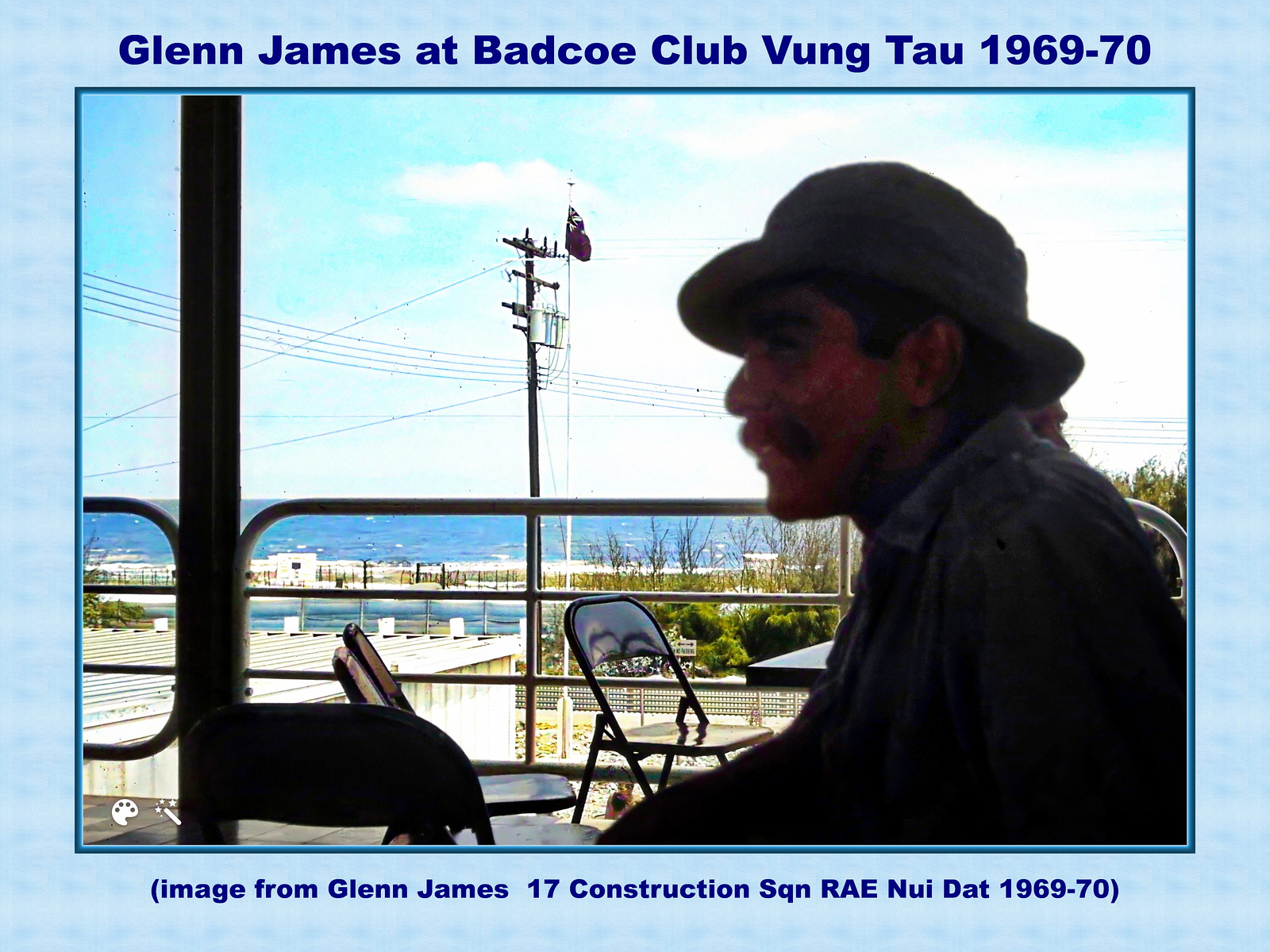The photograph, likely intended for a presentation or magazine, depicts a man seated outdoors on a patio. He is wearing a dark denim jacket and a black bolo cap. The man, who has a mustache and possibly glasses, is seated on a chair with another chair next to him. Across from him are a couple of folding chairs and a table. In the background, there is a steel fence leading to an area with green bushes, grass, and various buildings. You can see the ocean in the distance, under a partly cloudy sky, along with telephone poles and wires stretching across the scene. A red flag hangs from a flagpole near the railing. The photograph has a light blue border with blue text reading, "Glenn James at Bad Co. Club, Vontel, 1969-1970." The image is noted to be from Glenn James, 17, Construction Square, R-A-E-N-U-I-D-A-T, 1969-70.